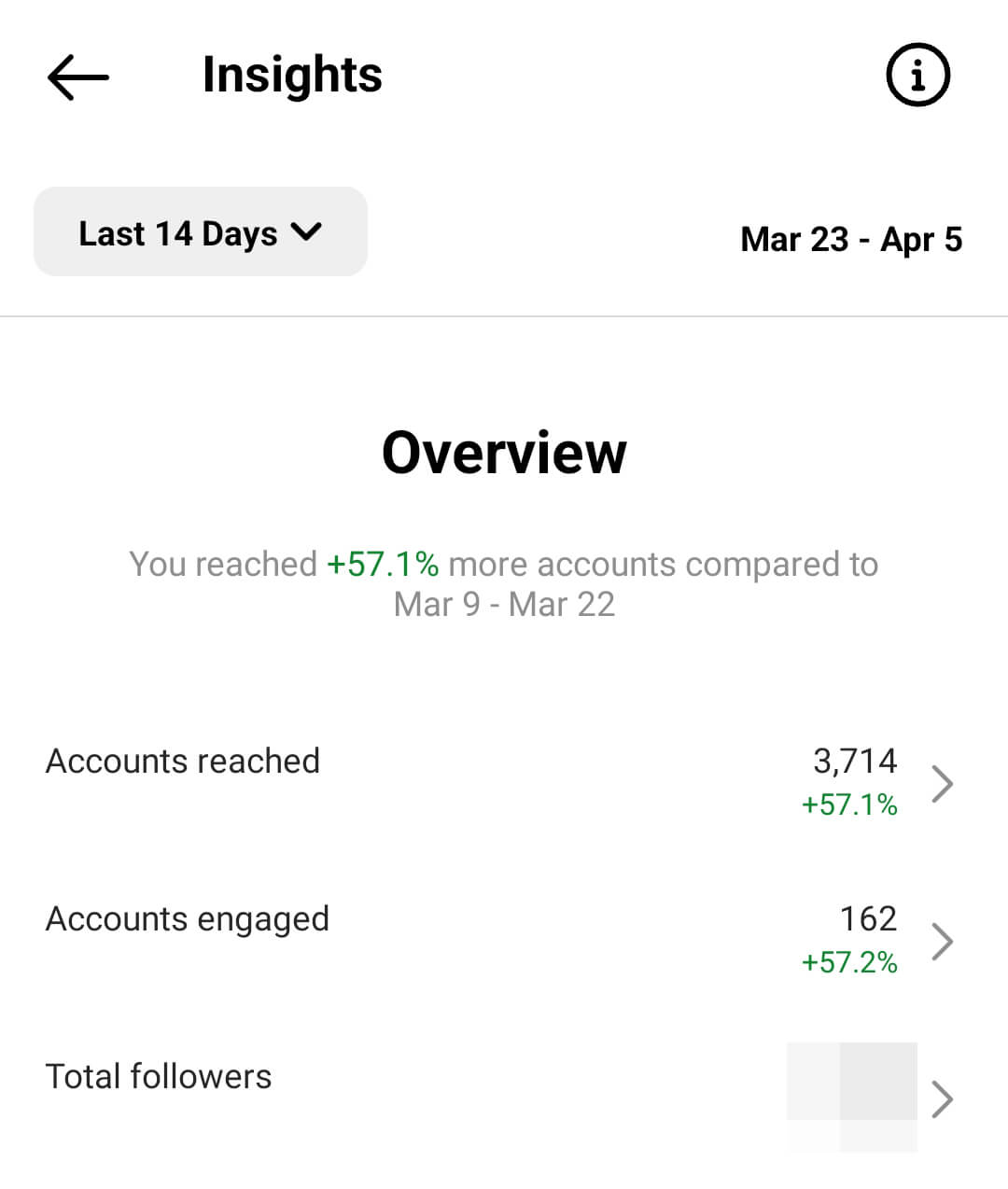**Caption:**

The image displays a detailed Insights summary for an account's performance from March 23rd through April 5th, compared to the previous period from March 9th through March 22nd. Positioned at the top left is the title 'Insights' with an arrow pointing left, and an eye icon enclosed in a circle on the right. 

In the top section, there is a dropdown menu labeled 'Last 14 Days,' and adjacent to it, the specified date range of 'March 23rd - April 5th'. A horizontal gray line runs across the middle, with the word 'Overview' bolded in black.

Below this line, the text states, "You reached +57.1% more accounts compared to March 9 through March 22," with the figure "+57.1%" highlighted in green and the remaining text in gray. 

Further details include:
- 'Accounts Reached' on the left side, indicating 3,714 accounts, again marked with the green "+57.1%" growth alongside a right arrow.
- 'Accounts Engaged' at 162, with a green "+57.2%" and a right arrow.
- 'Total Followers', which appears to have been obscured, presented in different shades of gray, followed by a right arrow.

The image features a predominantly white background with black, gray, and green text, focusing solely on account performance metrics without specifying the type of account or engagement goals.